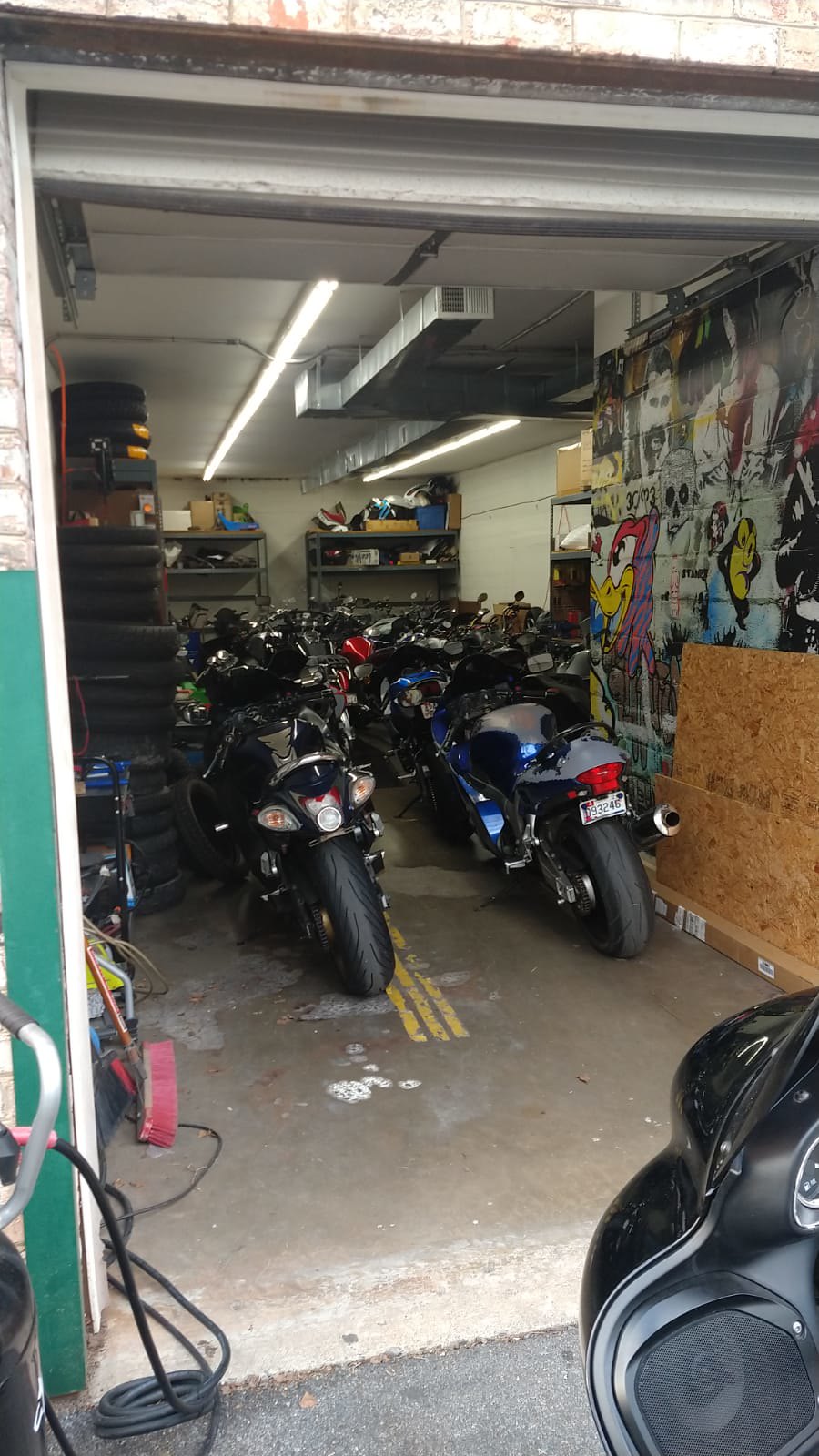The photograph depicts a narrow yet deep garage, densely packed with at least 15 motorcycles. In the foreground, the partial view of a motorcycle suggests the photographer may be seated on it. The garage, which can fit about two motorcycles across, has a distinctive yellow stripe down the middle resembling a road line. The right wall is adorned with vibrant graffiti featuring a variety of designs, including cartoonish characters like a duck with a yellow beak and a red face, and more realistic depictions of people. Leaning against this graffitied wall is a piece of plywood. The left wall has a large stack of motorcycle tires piled up to the ceiling and shelves at the far end loaded with various mechanical tools and supplies, with some more indistinct items and boxes. The ceiling is equipped with a long fluorescent light bulb and air-conditioning ductwork. Outside the garage, a green stripe is visible on the weathered white siding of the building, along with a brick facade. A barely discernible vehicle with a shiny auto-paint finish occupies the bottom right corner of the image.